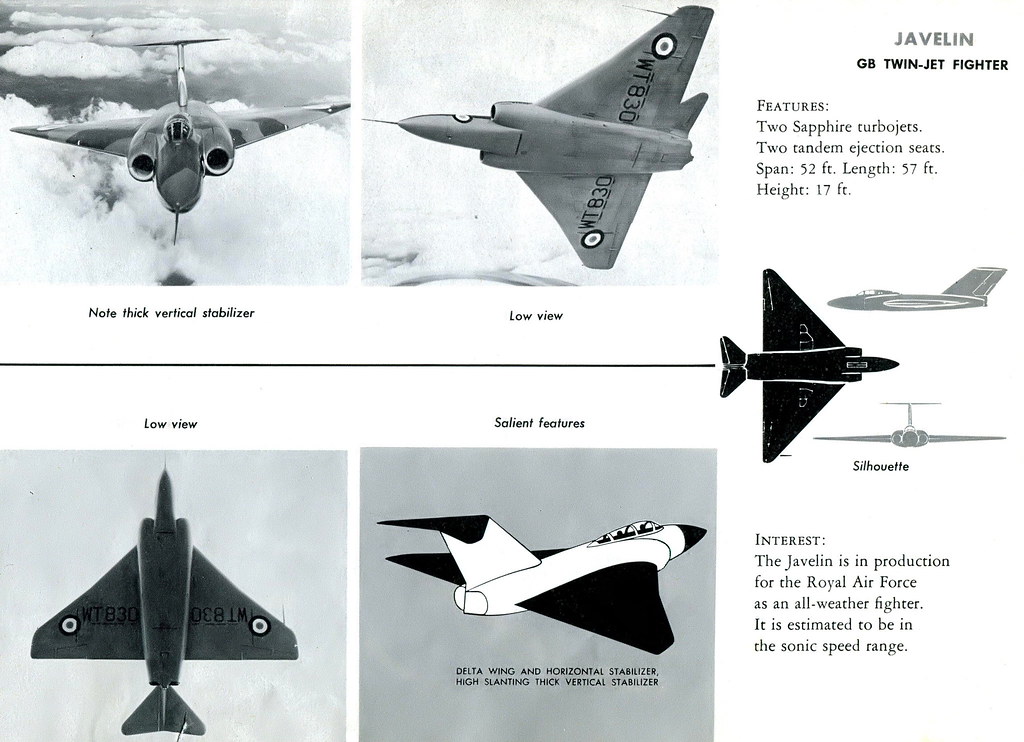This detailed black-and-white page showcases various renditions and photographs of the Javelin G8 Twin Jet Fighter, designed for the Royal Air Force as an all-weather fighter, estimated to operate in the sonic speed range. The layout is divided into four sections arranged in a two-by-two grid format. The top-left photograph presents a head-on view of the jet, highlighting the thick vertical stabilizer, whereas the top-right photo displays the fighter jet from a low, underside angle, indicated as "Low View." 

Below these, the bottom-left diagram offers another underside perspective labeled as "Low View," and the bottom-right illustration shows the jet at an upward diagonal angle towards the right, with the label "Salient Features." This section emphasizes the jet’s delta wing and horizontal stabilizer, accompanied by a high slanting thick vertical stabilizer.

On the upper right corner of the page, explicit specifications are listed: “Javelin, G8 Twin Jet Fighter, Features 2 Sapphire Turbo Jets, 2 Tandem Ejection Seats, Span 52 feet, Length 57 feet, Height 17 feet.” Additional notes describe the jet’s black wings, white body, and black-tipped nose with a glass window, alongside images of pilots. This detailed representation underscores the Javelin’s distinctive triangular design and strategic features.